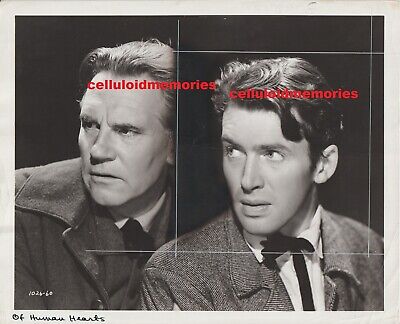The image is a black-and-white vintage photograph featuring headshots of two renowned actors of the period, Gregory Peck on the right and Walter Houston on the left. Both men are dressed in winter suits, with black ties and white shirts, and their hair combed backward in a slightly wavy style. The photograph is taken from the chest up and is set against a black background.

Peck and Houston are positioned side-by-side, facing the right side of the image but looking over their shoulders toward the top left. Their expressions convey surprise and slight worry, with wide-open eyes and alert gazes. The photograph appears old, with a visible white border framing the image.

Across both actors' foreheads, in bold red text, is the title "Celluloid Memories." A crop mark in a light white line is seen around Gregory Peck's portrait in the center. The bottom left margin bears a handwritten note in black ink, "Of Human Hearts," accompanied by a date written in white, "10-20-60." This carefully preserved moment captures an era and mood reflective of mid-20th-century cinema.